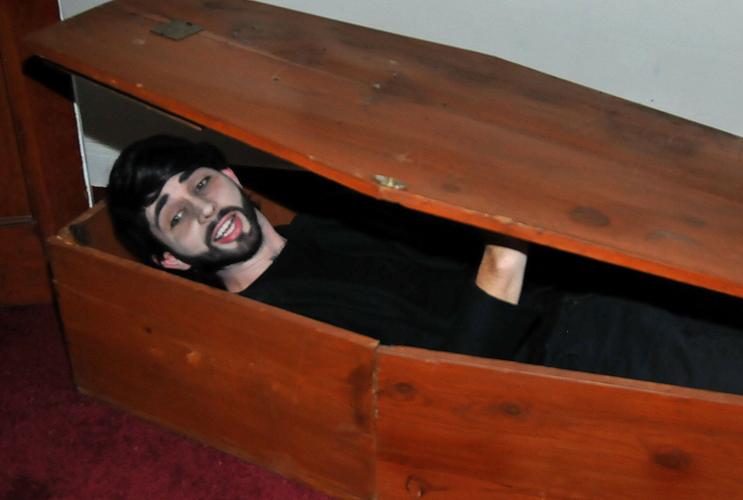This color photograph features a man inside a coffin with a glossy, reddish-orange wooden finish, set against a background of a white wall and deep mahogany wooden floor. The man, dressed in all black including a long-sleeved shirt and black pants, is lying inside the coffin and lifting the lid open with his arms, revealing himself with a slight smile on his face. His appearance is distinctly ghostly, with white powder makeup giving his complexion a pale, almost vampire-like look. He sports dark, slightly longer hair, which might be a wig, along with black eyebrows and a thick dark mustache and beard. His expression and pose suggest that he is playfully emerging from the coffin, adding an element of theatricality to the scene. No text or other elements are present in the photograph, making the man the sole focus as he looks out from the coffin.